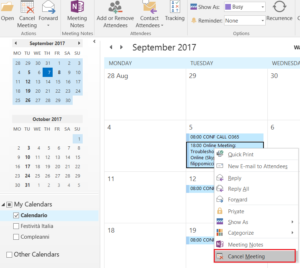The image depicts a menu within a calendar-type interface, which is somewhat difficult to read. The menu consists of a horizontal bar at the top of the image that stretches from left to right but is partially cut off on both sides. 

- The leftmost option on the bar is labeled “Open.”
- Following that are options labeled “Cancel Meeting,” “Forward,” and “Meeting Notes.”
- Next in line are options for “Add or Remove Attendees,” “Contact Attendees,” and “Tracking.”
- Towards the right section of the same line, several boxes are visible along with a “Reoccurrence” button.

The bottom portion of the image, which occupies most of the space, is divided into two sections:

- The left section features a vertical menu displaying two calendars.
- The right section provides an enlarged view of the selected calendar, which is September 2017. Within this calendar, notes appear to be made specifically for the 5th of September.